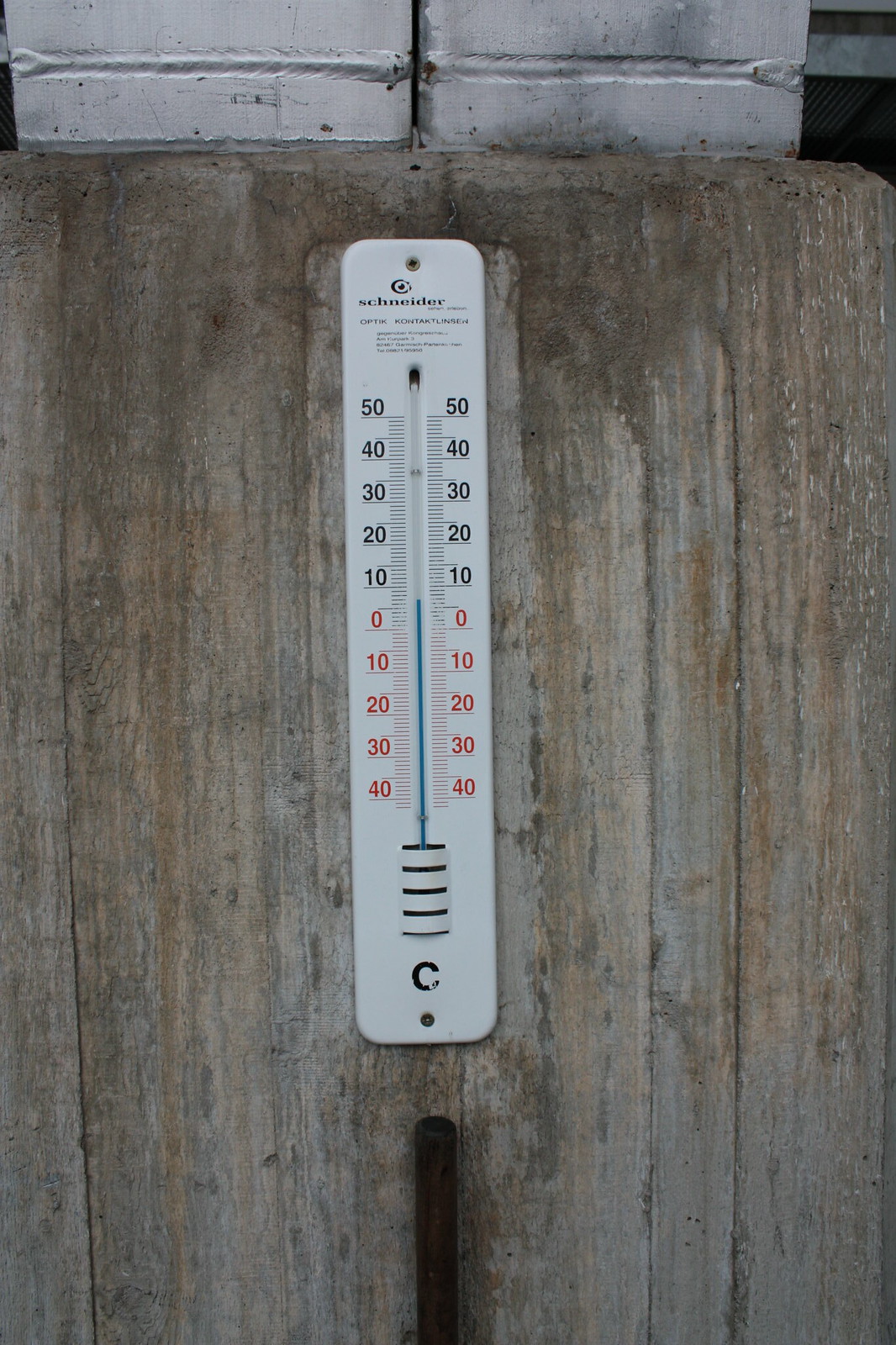The image features a plastic thermometer affixed to a piece of weathered wood. The wood appears dry and aged, with streaks of gray, tan, and brown running through it. At the top, the wood shows darker streaks, likely dirt that has run off from the adjacent white bricks above. These bricks are painted white and display patches of black, suggesting dirt or wear.

The thermometer, which is white, is secured to the wood with visible nails. It has a large "C" at the bottom, indicating it measures temperature in Celsius. The scale ranges from -40 degrees to 50 degrees, with negative temperatures marked in red and positive ones in black. The mercury inside the thermometer is dyed blue and currently indicates approximately 5 degrees Celsius.

Beneath the thermometer, a rounded wooden stick is visible, resembling the handle of a broom or mop. Black lines run underneath the mercury marker on the thermometer, providing a more precise measurement. All these elements come together to create a rustic and utilitarian scene.